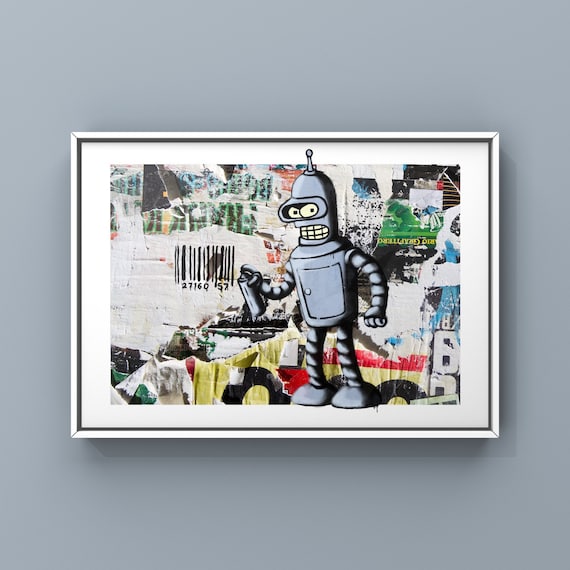This art installation features a dynamic painting of Bender from Futurama, prominently displayed against a plain gray wall. Encased in a white frame with a black interior rectangle, the artwork creates a striking contrast. The canvas itself appears crumpled and multidimensional, giving the illusion that Bender is popping out from a collage of torn newspaper pieces and various magazine clippings. These elements include discernible words and torn labels, contributing to a chaotic background.

Bender, rendered in shades of gray, stands out as the focal point. His expressive yellow eyes and wide-open mouth suggest a flustered or angry demeanor. In his left hand, he clutches a gray spray paint can, actively spraying a barcode streaked with brown or black. His right hand is clenched into a fist. Notable features like his yellow teeth and the accordion-like etches in his arms and legs add to the detailed depiction. His legs end in gray cylindrical boots, while the top of his head features a pointed antenna. The mixed-media background, combined with Bender's lively pose, makes for a visually compelling scene filled with movement and character.